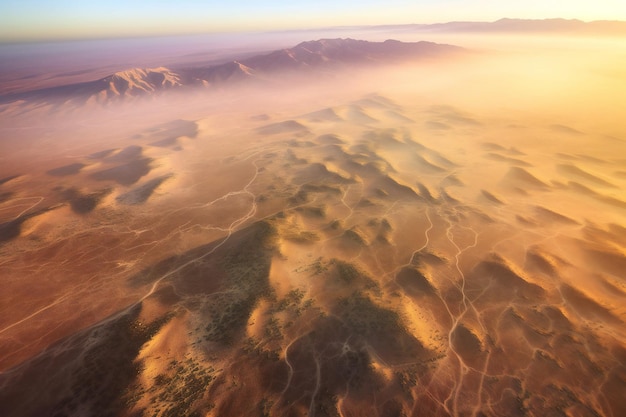This captivating color photograph, likely taken from an aerial perspective, presents a stunning outdoor scene where nature's elements come together harmoniously. The foreground is dominated by wind-sculpted snow dunes, which glow in golden and orange hues, possibly tinted by the low setting sun. These dunes vary in shape, creating an intricate, textured landscape reminiscent of desert sands. As the eye moves towards the background, the composition transitions to a majestic mountain range, partially shrouded in a misty, cloud-covered basin. The mountaintops pierce through this haze, highlighted by a purplish hue from the setting sun. Above, the sky features a crisp blue expanse with an orange band gracefully stretching across the horizon. The nuanced interplay of light and shadow throughout the image accentuates the depth and vastness of this breathtaking scene, making it a remarkable capture of nature's beauty.